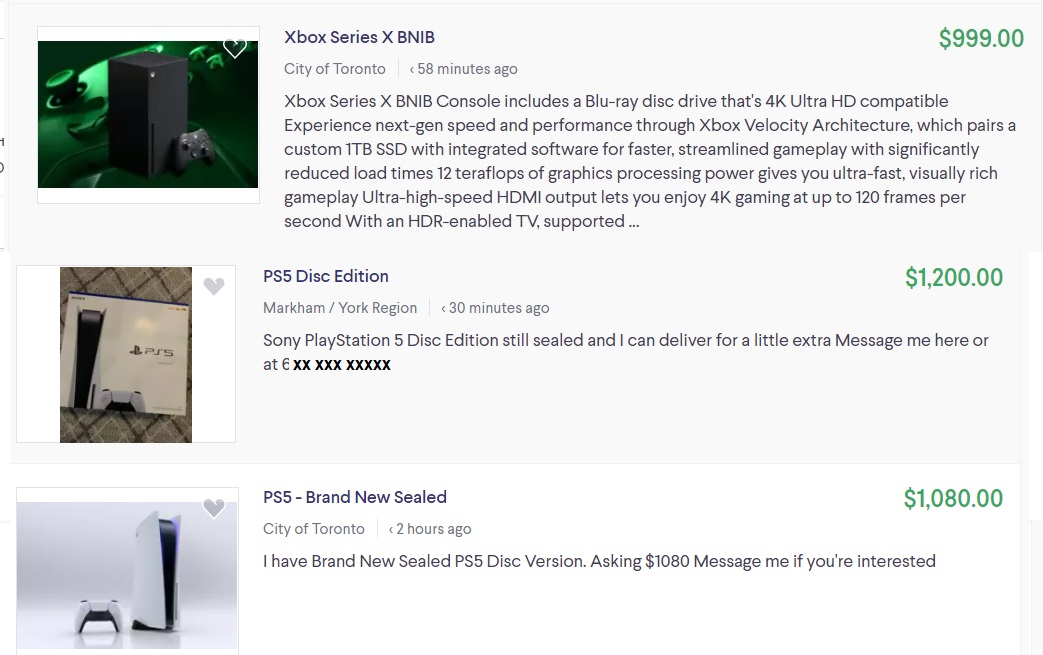The image consists of a screen capture showcasing three different advertisements for gaming consoles, each set against a white background with predominantly black text, and accentuated with a touch of green. The ads feature the following details:

1. **Xbox Series X Advertisement**:
   - **Image Description**: A black Xbox Series X console and a controller, set against a green background with game controller icons and a white heart symbol.
   - **Text Description**: "Xbox Series X BNIB, City of Toronto, 58 minutes ago." 
   - **Price**: "$999" in green.
   - **Details**: The listing mentions that the Xbox Series X is brand new in box (BNIB) and includes a 4K Ultra HD Blu-ray disc drive. It highlights the Xbox Velocity Architecture with a custom 1TB SSD, offering faster and streamlined gameplay with significantly reduced load times. The console features 12 teraflops of graphic processing power and ultra-high speed HDMI outputs, allowing 4K gaming at up to 120 frames per second with an HDR-enabled TV supported. The description cuts off mid-sentence.

2. **PlayStation 5 Advertisement (Markham/York Region)**:
   - **Image Description**: A white PlayStation 5 console, a white controller, and a white box with a thin blue strip at the top, accompanied by a grey heart symbol.
   - **Text Description**: "PS5 Disc Edition, Markham/York Region, 30 minutes ago."
   - **Price**: "$1200" in green.
   - **Details**: The Sony PlayStation 5 disc edition is described as still sealed, and the seller offers delivery for an additional fee. Contact details include a partially obscured phone number.

3. **PlayStation 5 Advertisement (City of Toronto)**:
   - **Image Description**: A white PlayStation 5 console and a controller against a stark white background, along with a grey heart symbol.
   - **Text Description**: "PS5 Brand New Sealed, City of Toronto, 2 hours ago."
   - **Price**: "$1080" in green.
   - **Details**: The ad mentions a brand new sealed PlayStation 5 disc version and invites interested parties to message for more information.

These detailed descriptions provide potential buyers with comprehensive information about each gaming console listing, including the product condition, price, and availability.